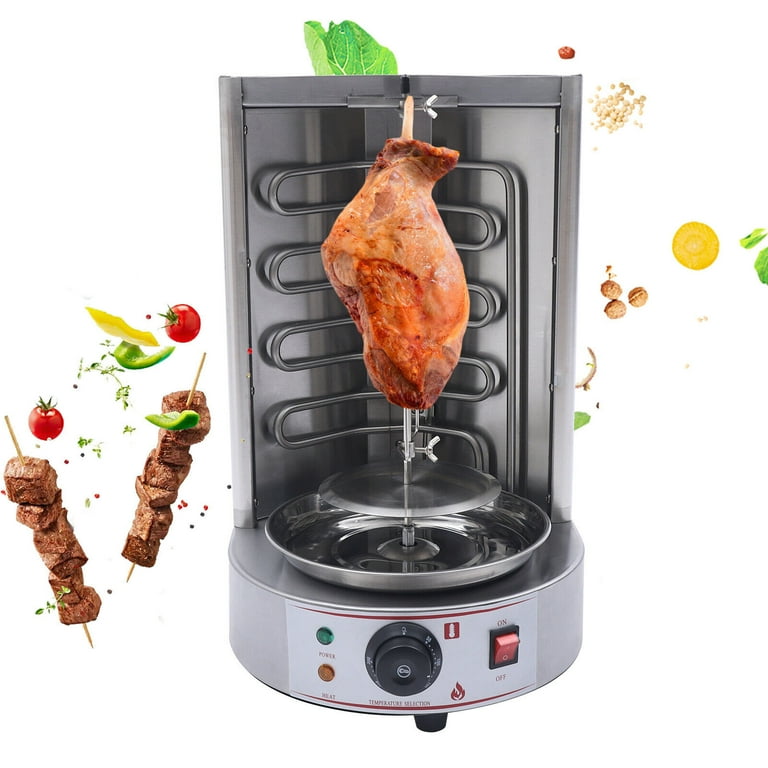In the image, a silver rotisserie cooker is prominently displayed with a piece of meat hanging vertically on a skewer inside. The front of the circular-shaped cooker is open, revealing silver heating coils in the back and a dial at the center bottom. To the right of the dial, there is a red on-off button, while to the left, small circular green and yellow power lights are visible. The cooker is set against a bright white background, scattered with illustrations of vegetables, including cherry tomatoes, green peppers, lettuce leaves, and yellow zucchini slices. To the left of the cooker, two shish kebabs laden with cubes of meat are depicted beside floating images of peppers and tomatoes.